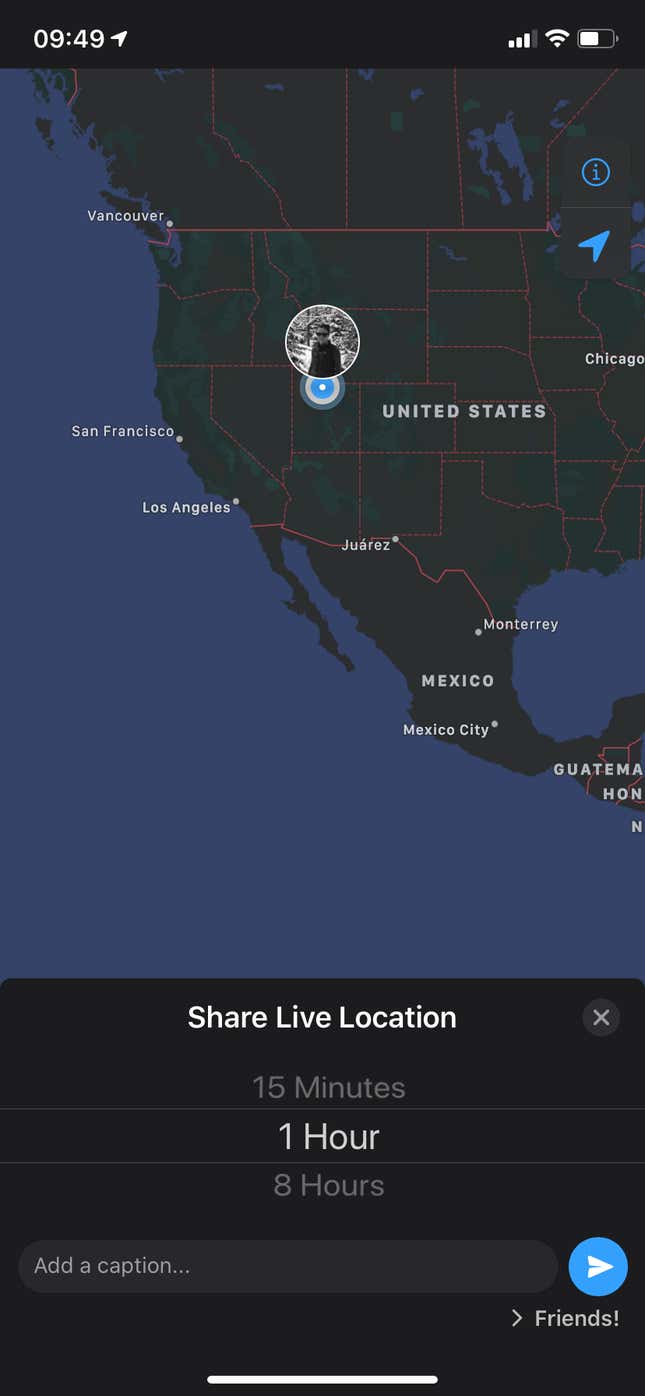The image is a screenshot from a mobile device, displaying a maps or location-sharing application. At the top of the screen, the status bar shows the time as 9:49 AM, along with signal strength, Wi-Fi connectivity, and battery icons. The central focus of the screen is a map featuring the United States, Mexico, and parts of Canada. Toward the center-left, a blue and gray circle with a white dot marks a specific location.

A black-and-white profile picture, presumably the user's, appears near the bottom left of the map. Additionally, a blue location icon is situated in the upper right section of the map, alongside an information button.

At the bottom of the screen, there is a black bar labeled "Share Live Location," presenting options to share the location for 15 minutes, 1 hour, or 8 hours. Below these options is a field to add a caption, paired with a blue "Send" button on the right.